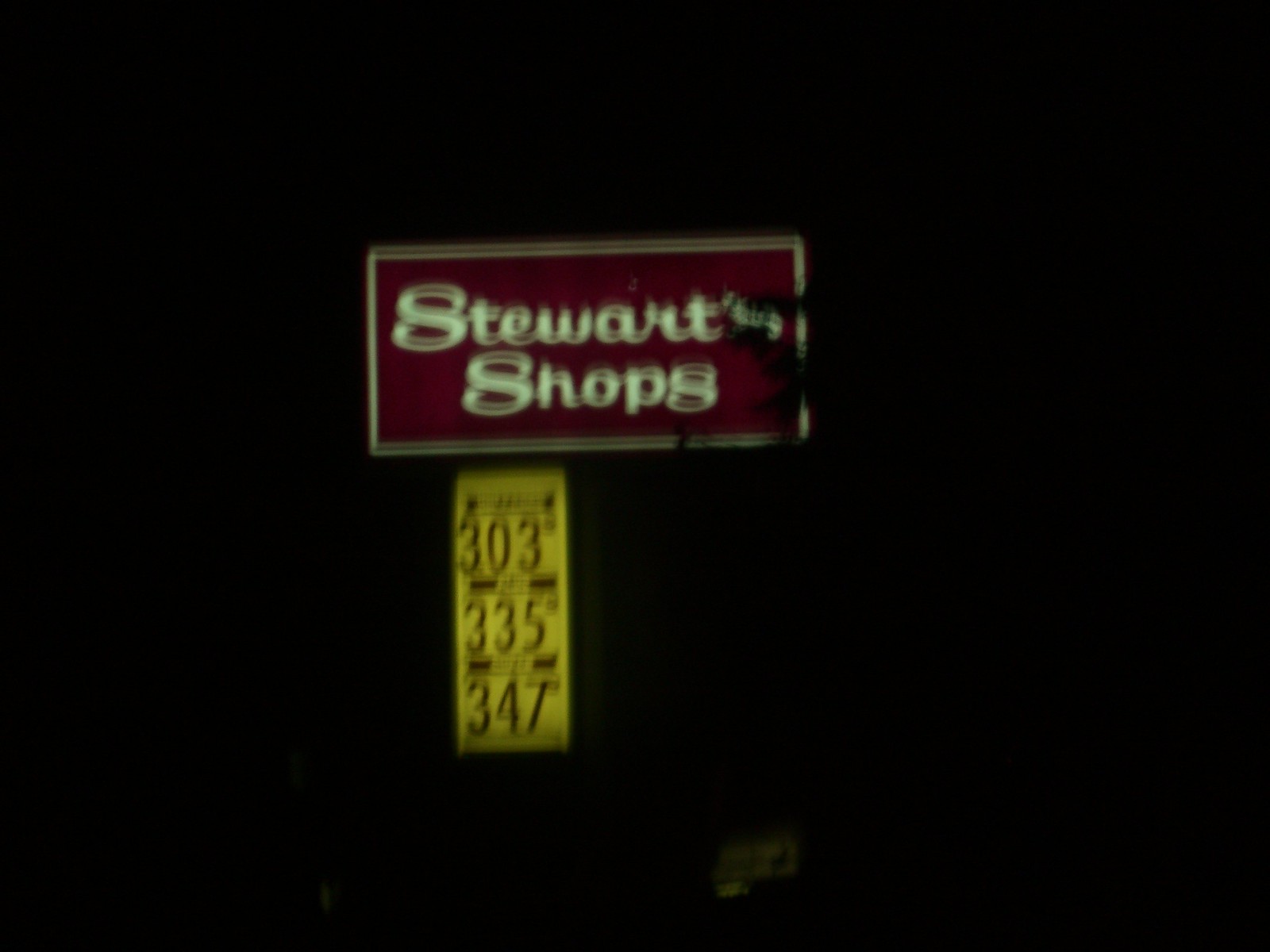This is a nighttime photograph of very low quality, characterized by its significant blurriness and predominantly black background. At the center of the image, two illuminated signs stand out. The first sign is a horizontal red rectangle with a thin white border. In an easy-to-read, slightly cursive script, it reads "Stewart's Shops." Beneath this, there is a vertical yellow sign with black text displaying gas prices. Due to the image's poor clarity, the labels for each price tier are unreadable, but the prices are discernible as follows: top price at 303, middle price at 335, and bottom price at 347.